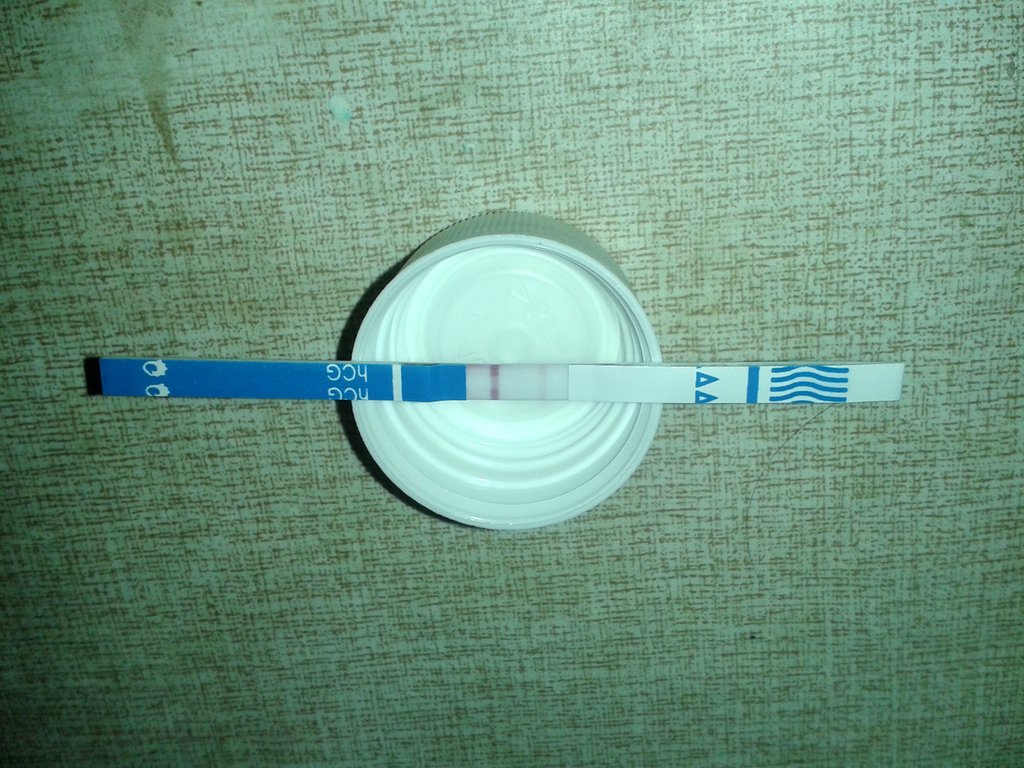The photograph features a single image focusing on a test strip that closely resembles a pregnancy test. The test strip is primarily blue and white, with bold white letters at the bottom that read "HCG." Near the top, the strip displays blue wavy lines, a blue dash, and two blue triangles. Centrally on the strip, there is a noticeable pink line alongside a very faint secondary pink line. Below these lines, there is a small white dash and the aforementioned "HCG" in white letters. At the very bottom of the strip, two small white characters are visible which interestingly resemble tiny feet. The strip is positioned atop a white, upside-down cap, within which some circular grooves are discernible. Both the strip and the cap rest on a soft surface featuring a combination of tan and white shades. A single brown human hair lies on this surface, which also has some tan-colored stains.